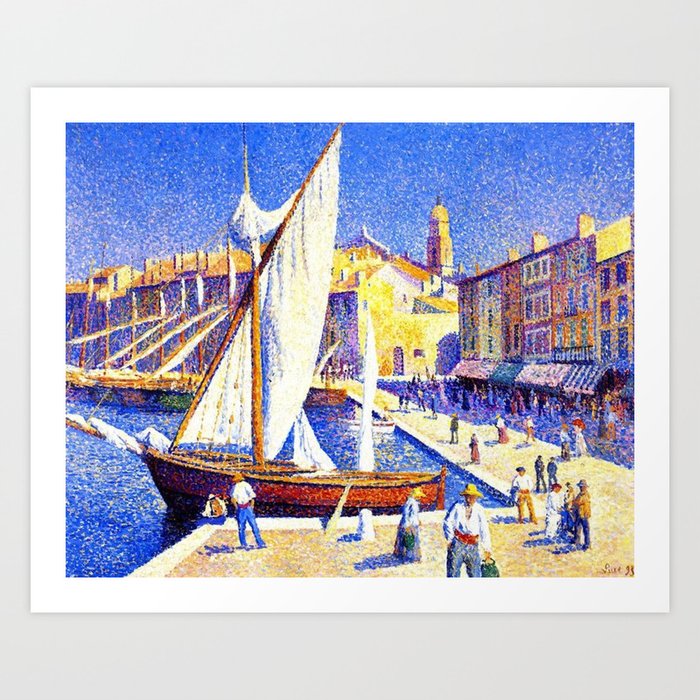The watercolor painting, framed with a white border, captures a bustling waterfront scene with a prominent sailboat moored at a dock in the center. This beautiful maritime image features a blue-hued background encompassing both the sky and calm waters. Surrounding the water is a lively boardwalk populated by faceless figures dressed as workers and tourists, their nondescript visages adding a touch of abstraction. The dock is flanked by an array of pastel-colored buildings, adorned with colorful awnings. Among these structures, some appear to house shops, while others might be residential with visible chimneys; a church tower and possibly a building under construction are discernible in the distance. The sailboat itself is accentuated by its brown hull and white sails, standing out as the focal point in this serene yet active waterfront tableau.